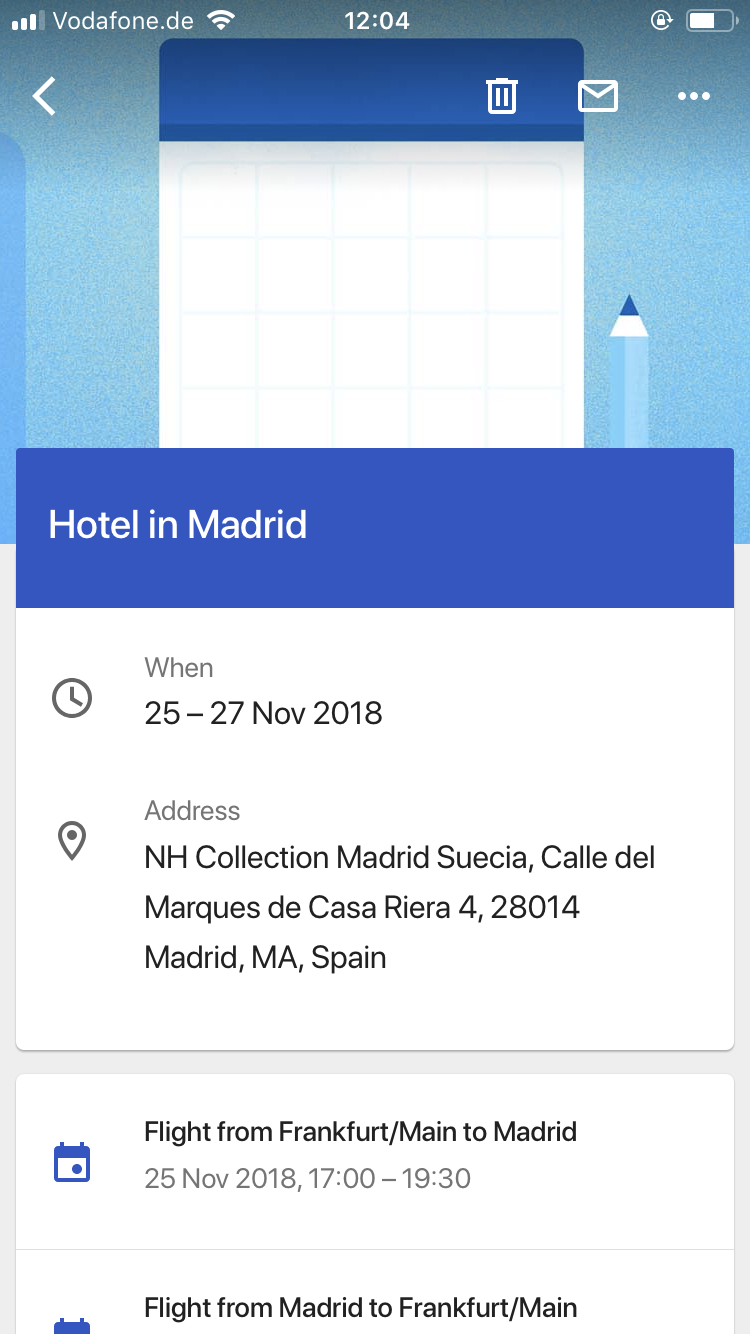The image is a portrait-mode screenshot of a mobile device interface, featuring multiple sections and travel details. 

At the very top, the status bar displays:
- On the upper left, it indicates the network provider as "Vodafone.de".
- The upper center shows the time, "12:04".
- The upper right depicts a battery icon that appears to be about half full.

Below the status bar, there is a toolbar that includes:
- A back arrow on the left.
- A trash can icon.
- An email icon.
- Three vertical dots for additional options.

The main background image appears to be a light blue blank calendar with a blue tab and a pencil, which has a light blue body and a dark blue nib.

A pop-up window occupies the central portion of the image with a blue header and white text that reads "Hotel in Madrid."

The pop-up contains detailed travel information divided into sections:
1. **When**: 
   - Dates: "25 to 27 November 2018"
   - Hotel: "NH Collection Madrid Suecia"
   - Address: "Calle del Marqués de Casa Riera, 4-28014, Madrid, MA, Spain."

2. **Flight from Frankfurt**:
   - Dates: "21st November to 25th November 2018"
   - Time: "17:00 to 19:30"
   - Destination: Madrid.

3. **Flight from Madrid to Frankfurt**:
   - Provides travel dates and returning flight.

Overall, the image showcases organized travel information about an upcoming trip to Madrid, including hotel stay and flight details.